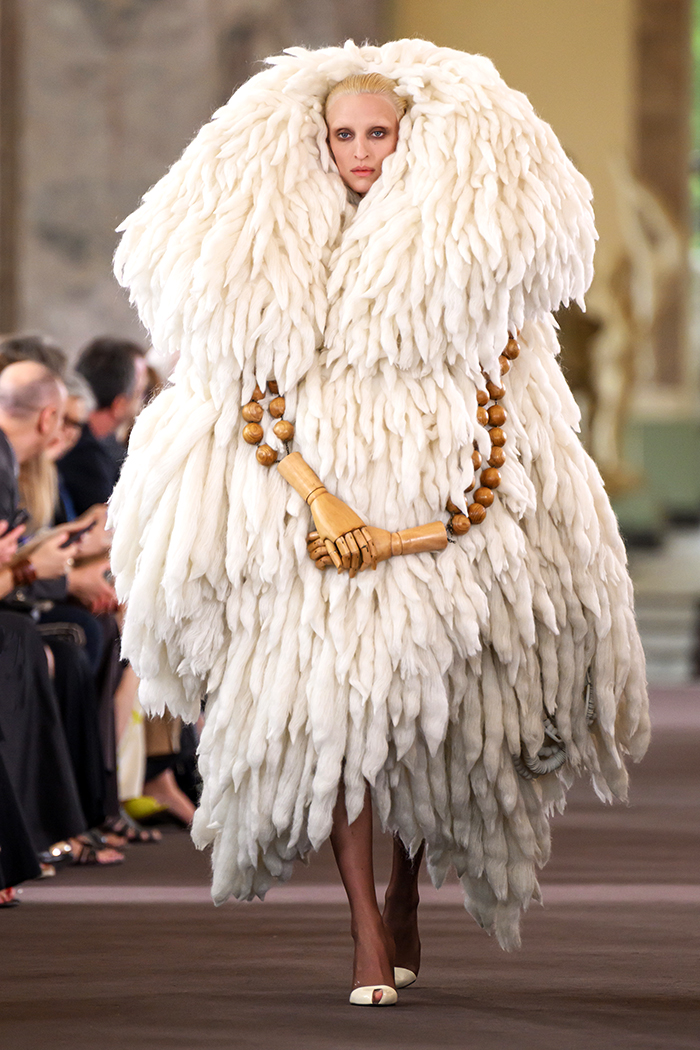The image captures a striking scene from a fashion runway, featuring a blonde, blue-eyed model with subtle makeup. She is adorned in a dramatic, feathery outfit resembling a cascade of white cotton braids that envelop her body in poofy layers, evoking an avian aesthetic. Her hair is slicked back and largely obscured by the outfit, save for her head. The ensemble includes unique accessories like wooden arms clasped together at the palms, hanging like a beaded necklace around her waist. The model completes her look with a pair of white shoes. The background reveals onlookers seated along the runway, their attention seemingly diverted to another part of the show. Dominant colors in the scene are white, brown, black, blue, and shiny brown.